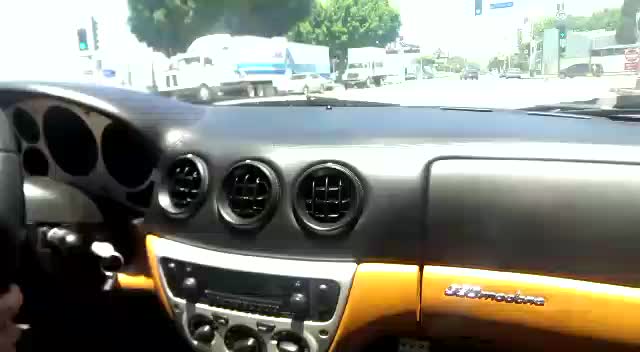The image captures the interior of a high-end, early 2000s vehicle, possibly a supercar. On the left side, a sleek steering wheel is prominently featured. Central to the dashboard are three air vents positioned in a horizontal layout at the bottom middle, framed by an elegant wood trim on the bottom right, exuding a classic luxury vibe. In the background outside the vehicle, various lights are visible, including a traffic light positioned at the top, hinting at a busy cityscape beyond the confines of the car.